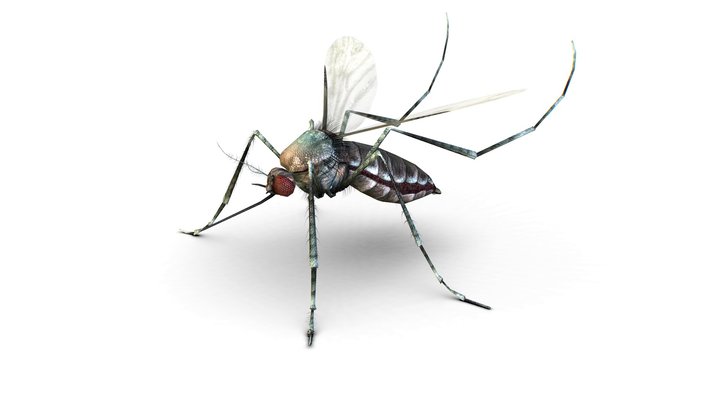This close-up side view image depicts a detailed rendering of a mosquito, capturing its intricate features with remarkable clarity. The mosquito, positioned on a transparent background, casts a distinct shadow below it. Its six long legs, notably light blue with individual hairs visible, show three positioned on the ground and two extending backward. One leg appears elevated on the left side, suggesting the insect is in mid-movement. The mosquito's small, spherical head is primarily red, adorned with large, compound eyes that have a textured appearance, akin to many small bumps. Its head also sports tiny antennae with delicate feelers.

The mosquito's round body exhibits white accents and a subtle shiny sheen at the top. The abdomen, a mix of gray and black, features beige at the bottom and light blue near the top. Strikingly translucent wings, displaying a delicate blend of gray lines, fan out from its sides—one fully visible on the left and the right partially due to its downward angle. The image’s artistic rendering enhances these physical details, making each feature pop against the transparent background.